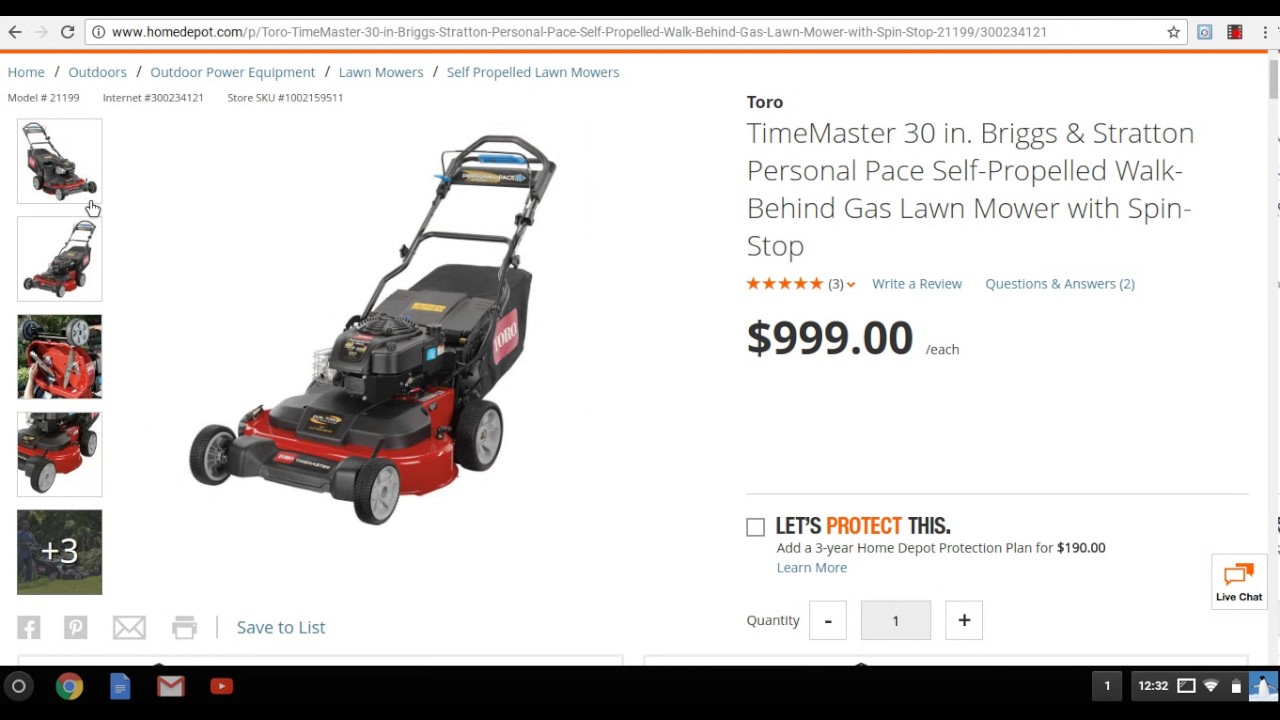A detailed screenshot from a laptop displays the Home Depot website featuring a lawnmower for sale. The specific product is the Toro TimeMaster 30-inch mower with a Briggs and Stratton engine, featuring personal pace technology, self-propulsion, and a spin-stop function. It is priced at $999.00. The product has three customer reviews, all rated at five stars, and there are two answered questions listed. The website’s URL, visible and lengthy, suggests the user has navigated through multiple products. The screen shows the person’s taskbar at the bottom with icons for Chrome, Google Docs, Gmail, YouTube, and a penguin icon likely for a Linux-based application. The Home Depot page has a plain design with a white background accented by signature orange elements. At the bottom right corner is a chatbot option. The product image currently displayed shows the lawnmower at an angle, highlighting its red base and black upper components. Seven thumbnail images in total are presented for the user to view.